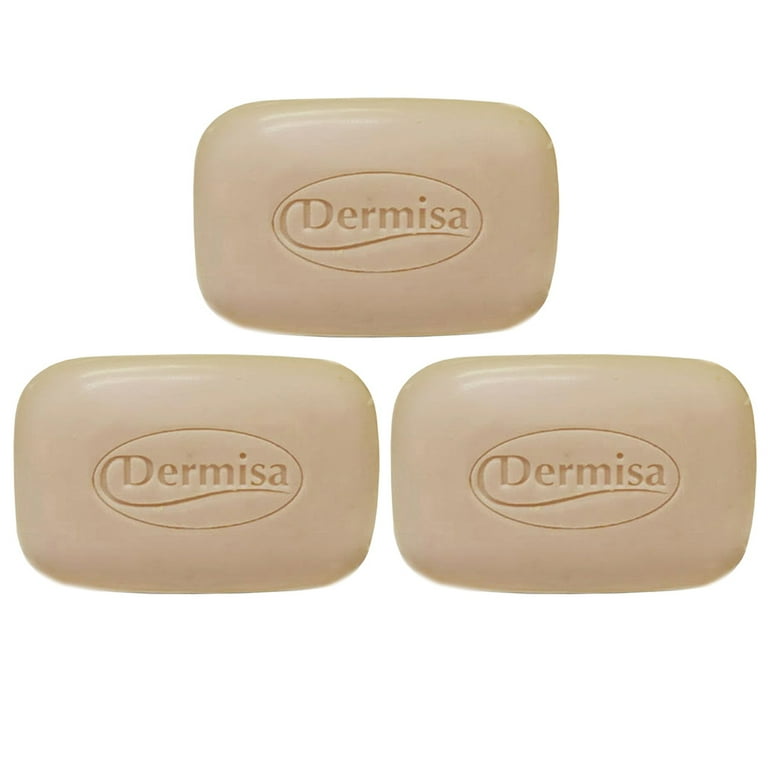The image features a set of three identical bars of soap against a white background. Each bar is a darker yellow, almost brownish color, and prominently displays the brand name "Dermisa" in capital letters. The logo's distinct design includes a red or white underline that sweeps from the left side of the capitalized 'D', creating a ribbon-like effect. Surrounding the "Dermisa" text is an oval frame, which is encompassed by a rounded rectangular border. The bars are arranged to face forward, emphasizing the brand logo in a basic, yet noticeable font. This image appears to be a stock photograph showcasing the Dermisa soap brand.